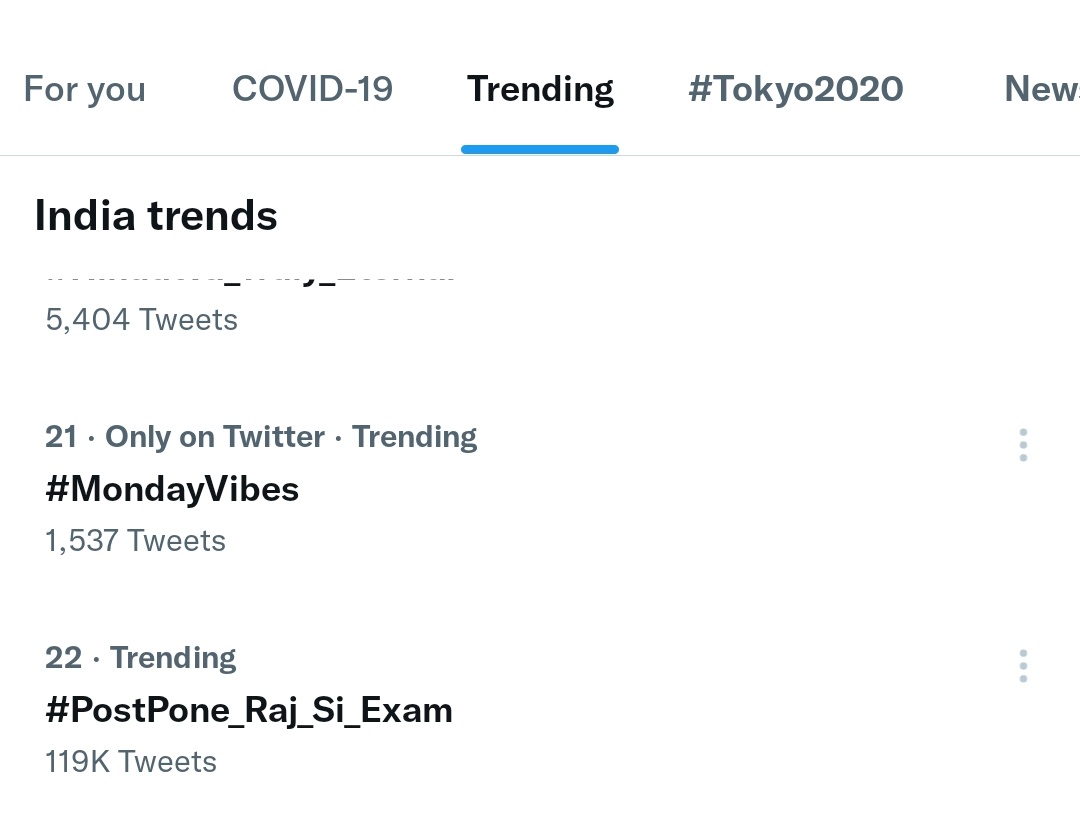Detailed Caption: 

This is a screenshot of an old Twitter interface, likely from the year 2020, during the COVID-19 pandemic and Tokyo Olympics. At the top of the screenshot, the "For you" tab is visible along with several clickable options, including "COVID-19," "Trending," and "Trending" is highlighted, indicating it has been selected. Below this, the hashtag "#Tokyo2020" followed by the label "New" can be seen.

Under the "Trending" section, there's a subheading titled "India trends," although the specific trending topic for India has been obscured. This section also notes that there are 5,404 tweets associated with the blocked-out trend. Further down, there's an entry numbered "21," labeled "Only on Twitter," featuring the trending hashtag "#MondayVibes" with 1,537 tweets.  

Following that is another trend numbered "22," with the hashtag "#PostponeRajCExam" and a significant count of 119K tweets. The rest of the image is blank, and on the right side, there are three small dots indicating additional options or trends that can be viewed. This sparse and slightly obfuscated screenshot captures a moment on Twitter during the rich and tumultuous events of 2020. There are no images, only text, capturing a historical snippet of the social media platform.